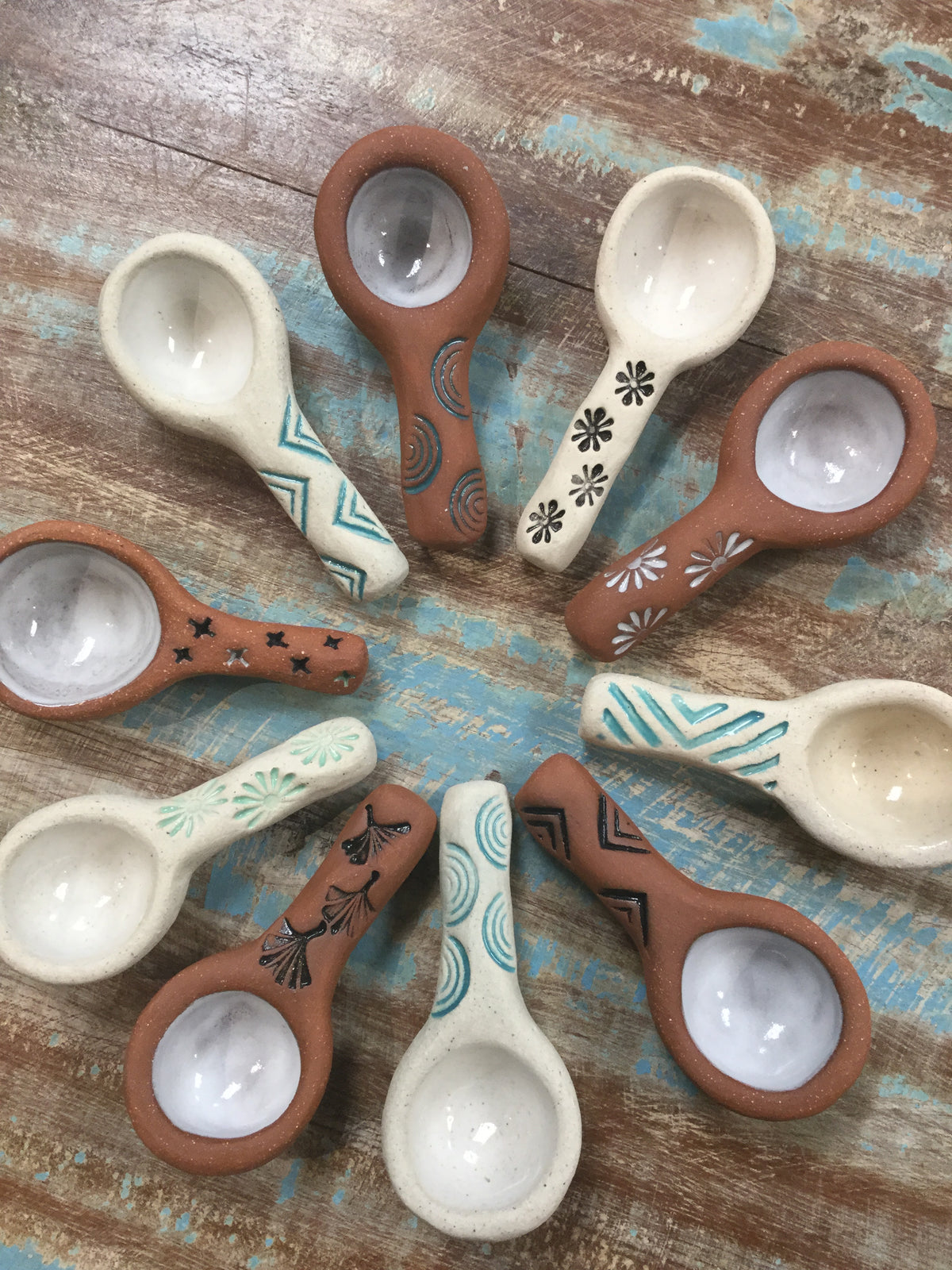This vibrant color photograph captures an exquisite arrangement of several small pottery spoons meticulously placed in a circular formation on a uniquely textured surface composed of distressed brown and blue wooden planks. Each spoon, characterized by its short handle and white bowl, showcases a harmonious blend of earth tones, with handles in various shades of brown and white. The artistry of the spoons is highlighted by the intricate decorative elements adorning their handles, featuring an array of lines, geometric shapes, and floral motifs. The image, oriented vertically, allows for a detailed view of the nuanced craftsmanship and aesthetic appeal of the spoons, creating a visually engaging and serene composition devoid of any text, people, or natural elements like plants, flowers, or trees.